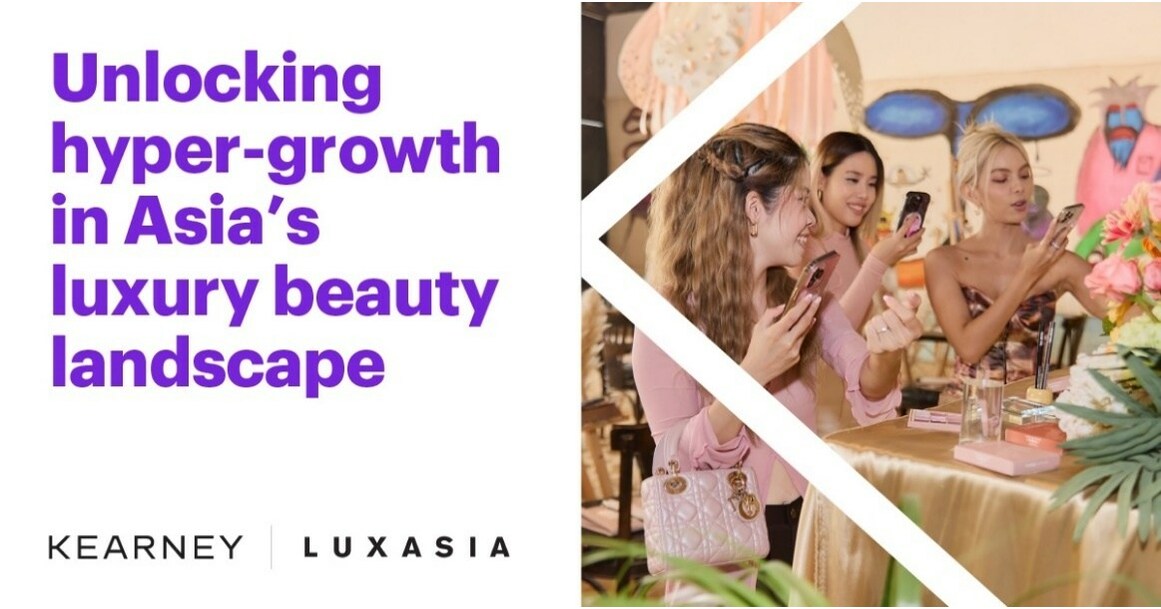In this image, we see an ad with text on the left and a photo on the right. The left side features a white background with the text "Unlocking Hyper-Growth in Asia's Luxury Beauty Landscape" in purple, and "Kearney" followed by "Luxasia" in black bold text at the bottom. Between these text sections, there is a line separating them.

On the right side, the photo showcases a lively scene of three young Asian women, likely in their twenties, at a stylish party. They're seated at an elegantly set table adorned with flowers and various beauty products. The women, all dressed in fashionable outfits, are capturing moments with their phones. The woman on the left has light brown braided hair, wears a pink top, and carries a pearlescent Dior Lady Dior bag, making a heart gesture with her index finger and thumb. The woman in the middle sports a pink long-sleeve top with her brunette hair down, while the woman on the right, with her hair tied up and makeup in a pinkish hue, dons a brownish strapless corset top. The background is vibrant, filled with blues, pinks, and other colors, reflecting the youthful and exuberant ambiance of the event.